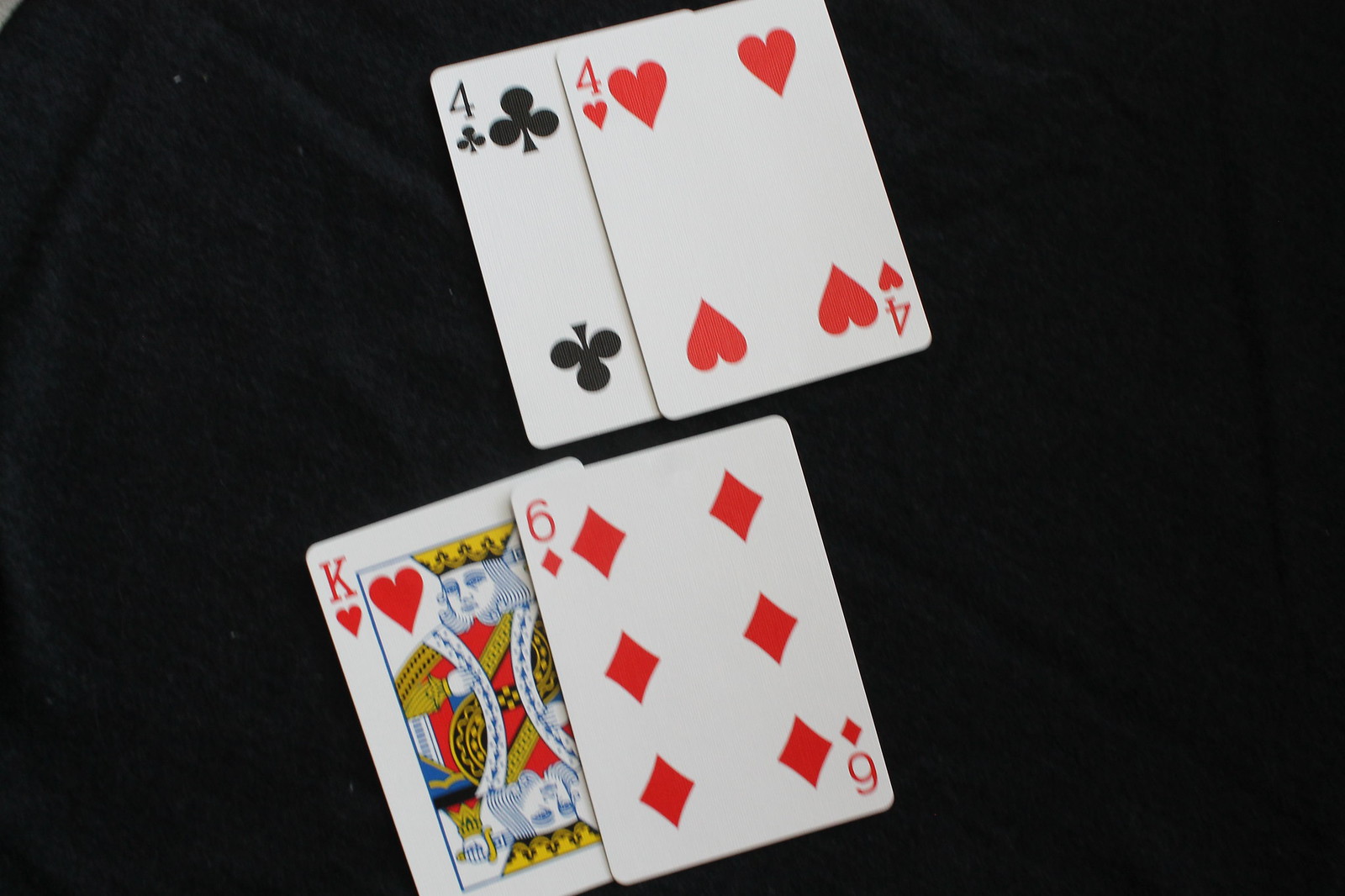In the foreground of the image, four playing cards are arranged in two overlapping rows. The top row features the four of clubs partially covered by the four of hearts, while the bottom row shows the king of hearts slightly overlaid by the six of diamonds. The cards are displayed face-up, revealing their values and suits, rather than their decorative backs. They are placed at a slight angle, with the bottom edges tilted approximately 15 degrees to the right.

The playing cards rest on what appears to be a piece of black cloth, adding a rich, contrasting background to the composition. In the upper left-hand corner of the image, there is a small, visible fragment of a white cloth or another object, offering a subtle contrast to the predominantly dark background.

The cards themselves appear to be fairly new, exhibiting minimal signs of wear or damage, maintaining a crisp and clean appearance.